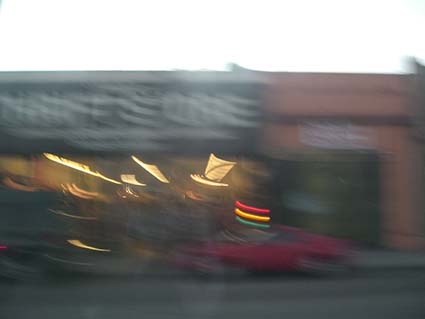A highly blurred photograph capturing the façade of two adjacent storefronts is shown. The left storefront features a dark blue banner with partially legible text hinting at "Thrift," and has large glass windows. Adjacent to it on the right is a brick building decorated with an American flag banner. In the foreground, there is a vividly colored red car. The lights in the image appear extremely bright and doubled, adding to the overall blur. Prominently in the frame, the hazy lights of a traffic signal display a sequential band of 3D colored lights: red at the top, followed by yellow, and then green.